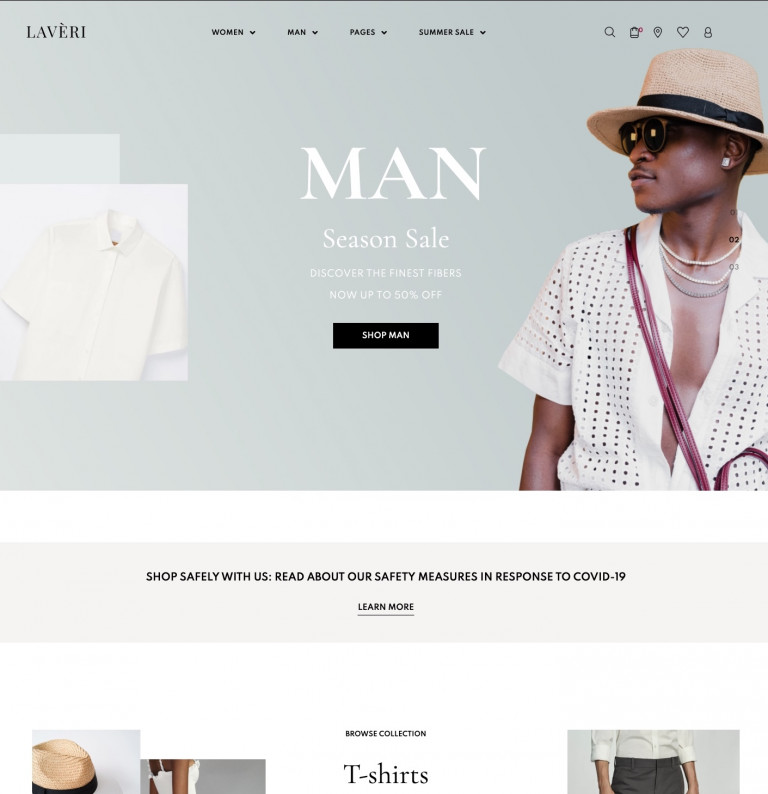The image is a vertically-oriented, slightly rectangular screenshot from a company webpage belonging to "LEVERI" (spelled L-A-V-E-R-I in capital letters), prominently displayed in the upper left corner. Along the center of the page horizontally, there are drop-down menu options labeled "Women," "Men," "Pages," and "Summer Sale." In the upper right corner, a series of icons are visible, representing functions such as Search, Items, Location, Favorites (Heart), and Profile (depicted as a little person).

Dominating the center of the webpage, bold white text in all-caps reads "MAN." Beneath this title, in a smaller combination of capital and lowercase letters, the text announces a "Seasonal Sale." Following this, another line reads "Discover the Finest Fibers Now Up to 50% Off," also in a smaller font. Below these lines, a small black button with white text labeled "Shop Man" invites users to explore further.

On the left side of the central text, there is an image of a short-sleeved white button-up shirt. To the right of the central text, an image features a black man wearing a white shirt with vertical columns of maroon spots, with the buttons left undone, revealing a portion of his chest. He is also wearing sunglasses and a tan hat adorned with a black ribbon around its base, as he gazes towards the left of the frame.